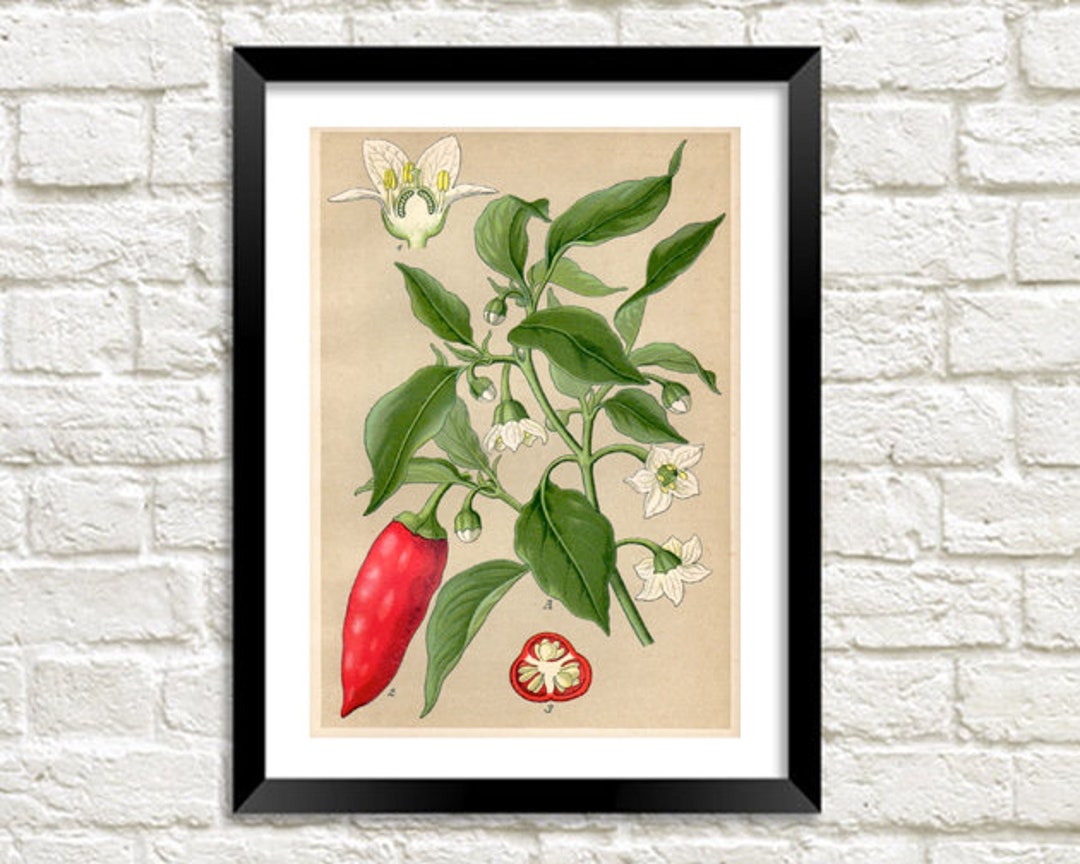The image depicts a detailed painting hung on a white brick-textured wall. The painting is enclosed in a black frame with a white mat around the image. The central subject of the artwork is a red pepper growing from a green, vine-like plant with large, pointed green leaves. The plant also features white flowers, characterized by green centers and yellow-tipped stamens. In the upper left corner of the painting, a single white flower is depicted more prominently, showcasing its intricate details with yellow buds emerging from the center. At the bottom of the painting, there is a cross-sectional view of the red pepper, revealing its interior structure. Additionally, various elements within the artwork are labeled, such as a leaf marked with 'A,' the whole pepper with '4,' and the sliced pepper at the bottom labeled '3.' The overall scene is bright and clear, accentuated by the natural lighting, giving a vivid and detailed portrayal of the botanical subject matter.